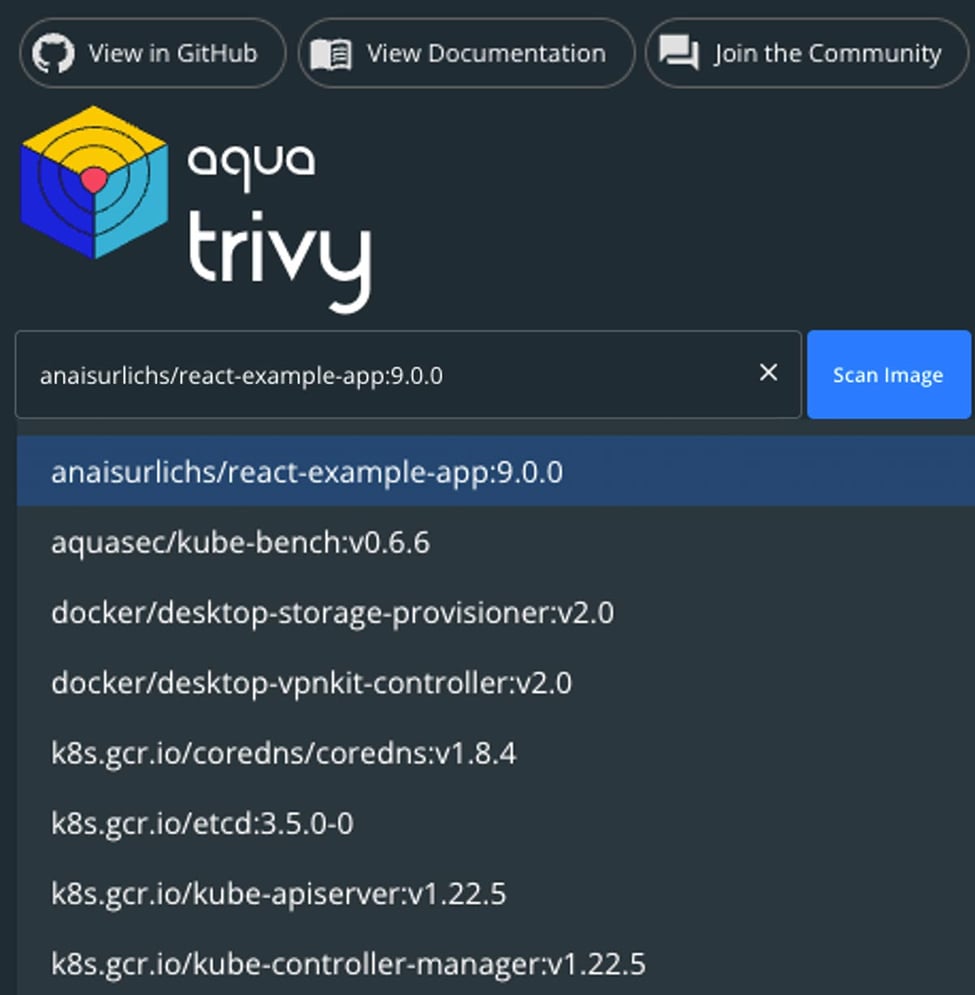In this image, we see a dark gray or deep blue website interface, reminiscent of GitHub's layout, filled with search results related to software downloads or image searches. At the top of the webpage, three buttons are prominently displayed: "View on GitHub" with the GitHub logo, "View Documentation" with a book icon, and "Join the Community" with overlapping comment icons. Below these buttons, on the left-hand side, is the title "Aqua Trivia" presented in a sharp, striking font, accompanied by a hexagonal logo featuring yellow, blue, and red colors.

Directly beneath the title is a text field and a blue button labeled "Scan Image." Following this input section is a list of search results composed of various terms or addresses, potentially representing different apps. The specific search query used is "Anastolik-react-example-app: 9.0.0," which is also highlighted in a light blue box at the top of the results. The remaining results are similarly formatted, with a consistent, lighter gray background color that differs from the main backdrop.